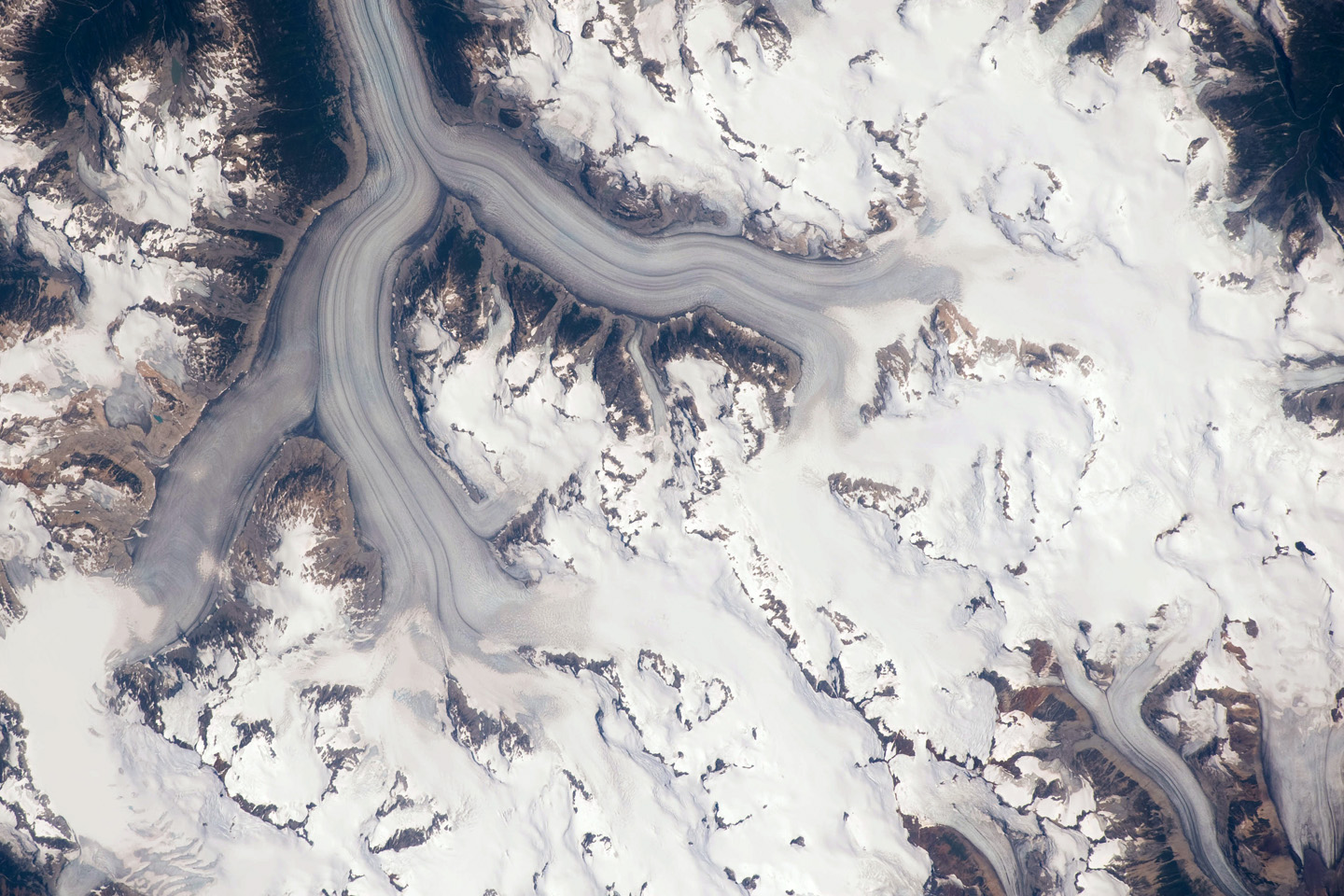This is a detailed, color satellite image of a mountaintop or rocky formation that is almost entirely covered in snow. The image, taken from space, highlights a deserted and unpopulated area without visible people or animals. The mountaintop features prominent peaks and jagged rocks, with predominantly white snow interspersed with patches of dark brown and gray stone. There are noticeable ridges and lines within the snowy expanse, resembling roads or waterways, particularly a faint gray jet stream-like formation that branches into a two-pronged fork at the top of the image and extends downward. Towards the top, a dark formation with a forked structure can be seen, giving an impression of a branch or waterway descending from the rocky summit amidst the predominantly snowy terrain.